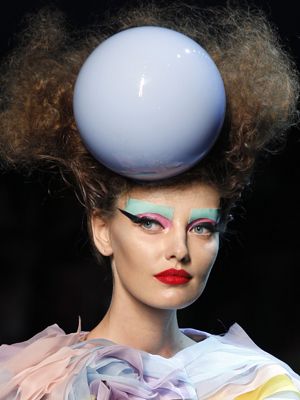This image features a photograph of a woman, presumably a high fashion model, positioned against an all-black backdrop. The composition captures her from the chest upwards, emphasizing her head and shoulders. The woman has a striking appearance with frizzy, curly dark brown hair that has been teased to stand upright reminiscent of the Bride of Frankenstein. Resting on top of her hair is an oversized, pale blue ball that appears to be affixed, serving as a focal point and adding to the avant-garde aesthetic.

Her makeup is bold and vivid: she wears bright red lipstick, dramatic black winged eyeliner extending nearly to her temples, and vibrant eyeshadow in shades of pink and blue. Her eyebrows are partially obscured by a teal square, contributing to the surreal quality of her look. The makeup is further accentuated by her poised, off-camera gaze.

The woman's attire consists of a pastel-colored top adorned with shades of orange, purple, blue, and yellow, though only her shoulders are visible. Overall, the photograph exudes a high-fashion, runway vibe due to its dramatic and unconventional elements.